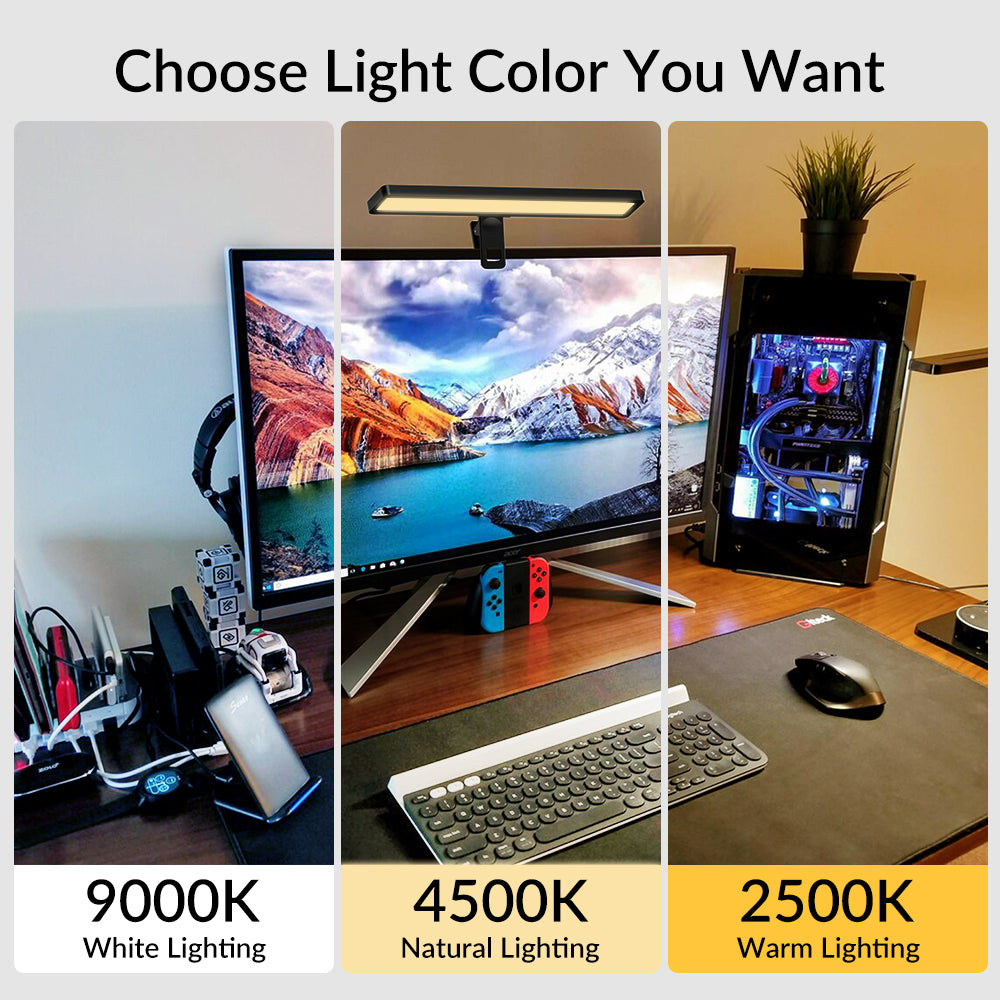The photograph showcases a desktop setup illuminated by three different types of lighting, emphasizing the message "Choose the light color you want" at the top. The image is divided into three vertical sections, each displaying a distinct lighting effect: the left section features 9000K white lighting, the center section has 4500K natural lighting, and the right section shows 2500K warm lighting. The desktop setup includes a screen, keyboard, and mouse placed on a brown table, surrounded by various electronic objects on either side. The 9000K white lighting imparts a stark, clinical feel similar to a hospital environment. In contrast, the 4500K natural lighting provides a more muted ambiance. The 2500K warm lighting emits a soft yellow glow, creating a homey and inviting atmosphere, giving the room a touch of class and warmth. The gray background further highlights the differences in the lighting effects.